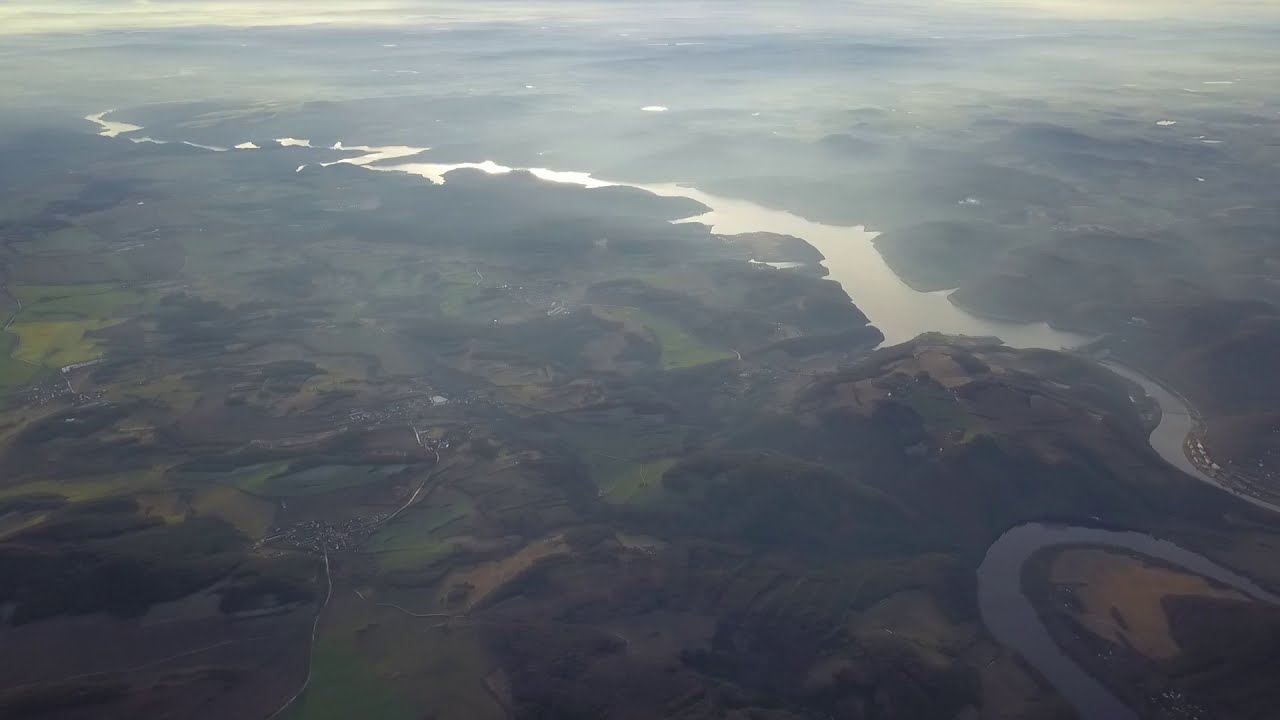The image is an aerial view taken from a very high altitude, most likely from a drone or aircraft, capturing a stunning, vast landscape of low-lying mountains and a long, winding river. The river, reflecting sunlight, snakes across the terrain from the bottom left to the top right, appearing to cut through the hills for several miles. The scene is somewhat hazy due to a layer of low-level clouds or mist, which partially obscures the finer details but contributes to the overall atmosphere. You can make out patches of greenery, suggesting dense vegetation, forestry, and possible farmland. There are hints of man-made structures like roads and possibly a dam leading to higher water levels in the valley. Near the bottom left of the image, you can see small dots indicating towns or houses, and there are areas that suggest circular or oval formations, possibly golf courses. The image evokes memories of rural regions like Appalachia in West Virginia, characterized by mountainous areas with rivers weaving through them.